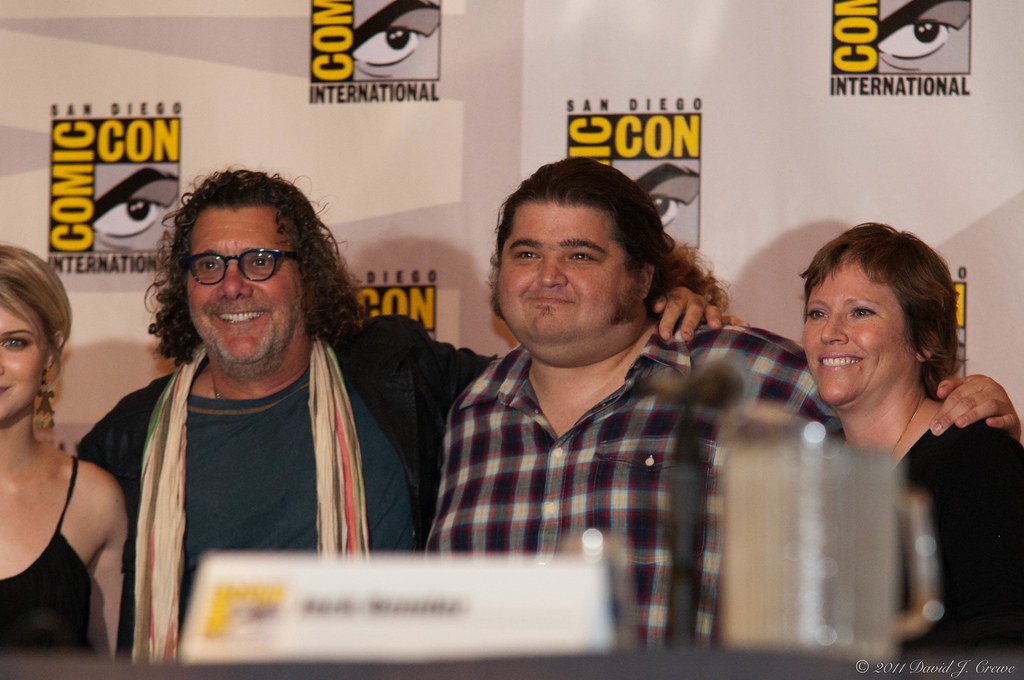In this image, four individuals are standing closely together with their arms around each other's shoulders, posing for a group photo. They are dressed casually and appear to be at an indoor setting, likely a convention. A white backdrop with a repeating logo for "San Diego Comic-Con International" in black and yellow is prominently displayed behind them. Though the people are mostly centered in the image, the person on the far left is slightly cropped off. Among them, an actress and a heavyset man with long hair from the TV show "Lost" are recognizable. There is a table partially visible at the bottom of the image, which holds a pitcher of water and an unreadable name tag. The background and environment suggest it is part of a press or fan event at the Comic-Con convention.